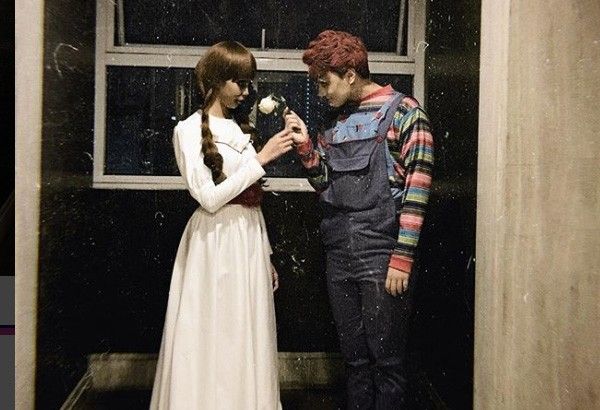The photograph captures a young couple, likely in their late teenage years or early 20s, standing in a dimly lit, narrow hallway with a window that appears pitch black, possibly indicating nighttime. The image has a vintage feel, with specks and dust suggesting it was taken with a film camera. The girl, who has long braided brown hair cascading to the small of her back and bangs, is wearing an ankle-length, flowing white dress that covers her from neck to wrists. She’s reaching out to accept a slightly wilted white rose from the boy, who has striking red hair and very pale skin, enhancing a somewhat eerie appearance. He is dressed in dark denim overalls with a front pocket, layered over a horizontally striped long-sleeve shirt featuring an array of vibrant colors including orange, black, green, blue, red, and pink. The couple bears a resemblance to characters resembling Chucky and his bride, adding a slightly theatrical, spooky touch to their appearance, possibly accentuated by makeup to make their skin look paler. The girl is tan and appears to be wearing a wig. The setting is further characterized by contrasting light wood and dark walls, adding depth to the backdrop of the couple’s interaction.